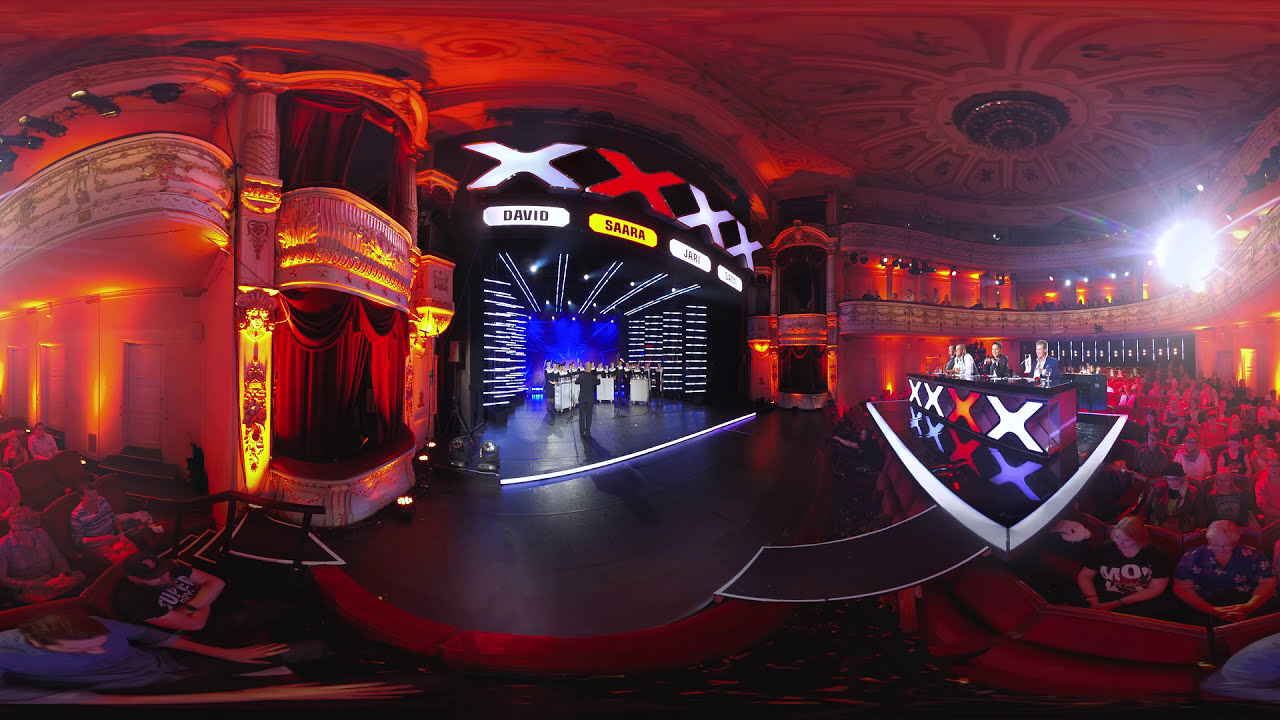The image depicts a live session of "The X Factor" talent show. The scene captures a theater-like venue filled with an audience seated in red chairs, extending to a balcony above. The audience is keenly observing the stage, where a choir of around 20 participants, dressed like nuns, perform under spotlights. To the right-center of the image, four judges can be seen seated at a desk, their names displayed above them. The names include David, Sarah, Jerry, and another that is partially obscured. Sarah's name is highlighted in yellow, with a red X indicating her disapproval of the performance. The ceiling of the venue is adorned with intricate designs, adding to the grandeur of the setting.